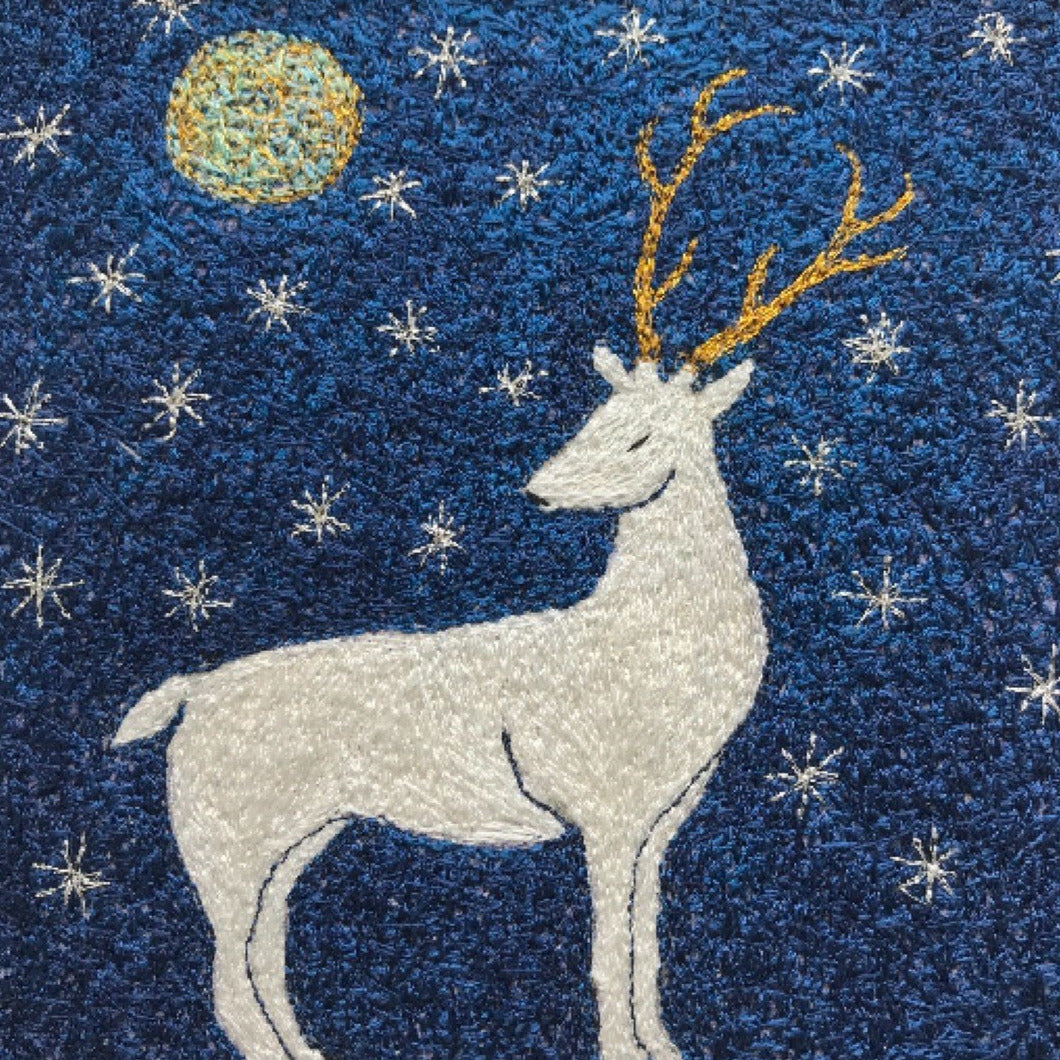This detailed and textured image captures a beautifully crafted white reindeer or stag with large golden antlers, showcased in a medium that resembles either a painting on carpet, needlepoint, or a woven quilt. The stag's body faces to the right, but its head turns almost completely back, gazing thoughtfully behind itself with a closed eye, suggesting a serene or contemplative state. Set against a richly textured, deep blue background with varying shades, the scene is adorned with numerous white stars, which add to its tranquil ambiance. The top left corner features a large, yellow moon that contributes to the mystical feel of the artwork. The piece's intricate darker line work accentuates the stag's legs and jawline, enhancing its lifelike appearance. Overall, the image exudes a peaceful, ethereal quality.